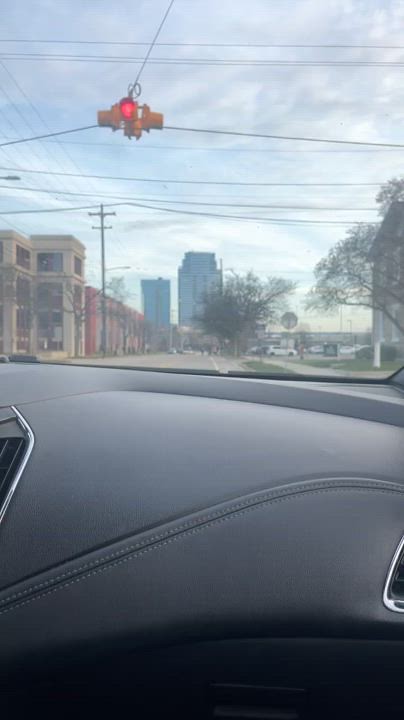The image captures an intricate scene from the interior of a car, showcasing a detailed urban environment through the windshield. The car is stopped at a four-way intersection with a red light facing it. The dashboard, a prominent feature in the foreground, is made of black leather with distinct hills and valleys, featuring two air conditioning vents trimmed in silver and displaying some angular stitching towards the center.

Beyond the windshield, a bustling cityscape unfolds. On the left side of the road, two- and three-story buildings stand tall, with red brick exteriors and beige frontscapes, while in the distance, towering office buildings made of glass and gray metal rise, some of them as tall as 20 stories. To the right, there is a car dealership and a parking lot. The road ahead is marked by a white line, and overhead, numerous wires crisscross the scene, beneath a sky thick with cloud cover. Branches with foliage from nearby trees also frame the view, adding a touch of nature to the urban setting. The other side of the street features a stop sign rather than a light, completing the busy yet organized city view.